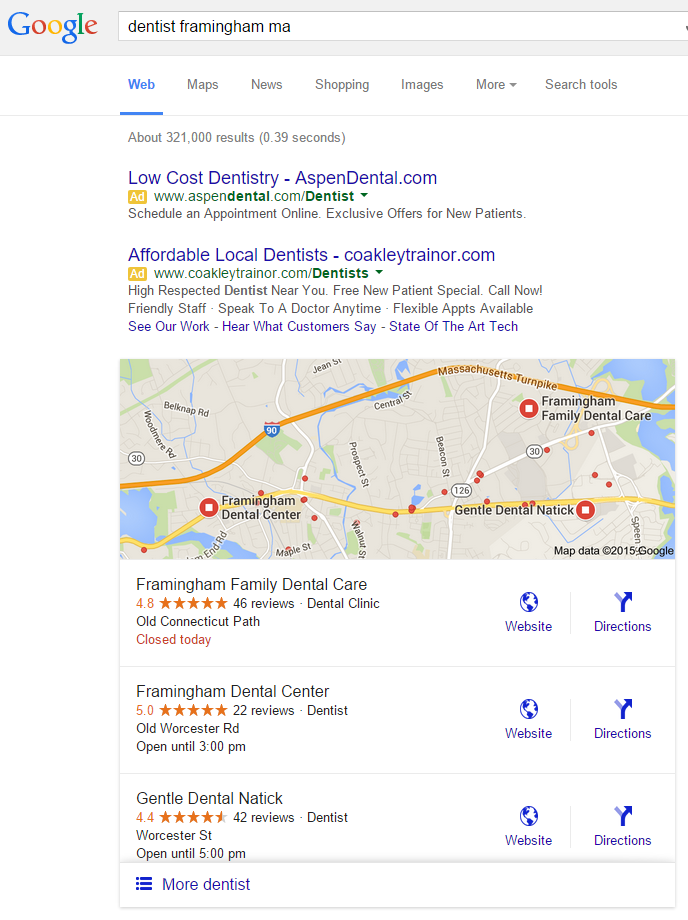The image depicts a Google search results page with a gray border across the top part of the background. On the left side of the border, the word "Google" is prominently displayed in its iconic multi-colored lettering: blue, red, yellow, blue, green, and red. Below the border is a white search box, partially cut off on the right side, with the search query "dentist Framingham, MA" typed in black text.

The main content area has a white background and features various tabs just below the search box. The first tab is highlighted in blue text with an underline, indicating it is selected. It reads "All," while other tabs like "Maps," "News," "Shopping," "Images," and "More" are displayed in dark gray.

Below the tabs, a gray line separates the tab area from the search results, with text that reads "About 321,000 results (0.39 seconds)" in a lighter gray font. The first search result is marked by a purple-blue hyperlink that says "LocalDentist.com," followed by a yellow rectangle with the word "Ad" in white. The green text reads "www.localdentist.com," followed by a description in black text reading, "Schedule an appointment online. Exclusive offers for new patients."

The second result is similarly formatted, with a purplish-blue hyperlink to "Affordable Local Dentists - CoakleyTrainer.com," denoted by another "Ad" label in yellow. The green text states, "www.coakleytrainer.com/dentist," with a black text description: "Highly respected dentists. New patient special - Call now! Friendly staff, speak to a doctor anytime, flexible appointments."

Following the text ads is a map section, showing locations such as "Framingham Dental Center" and "Gentle Dental." Accompanying links are provided for these places, including "Website" and "Directions" in blue text, along with additional practice information.